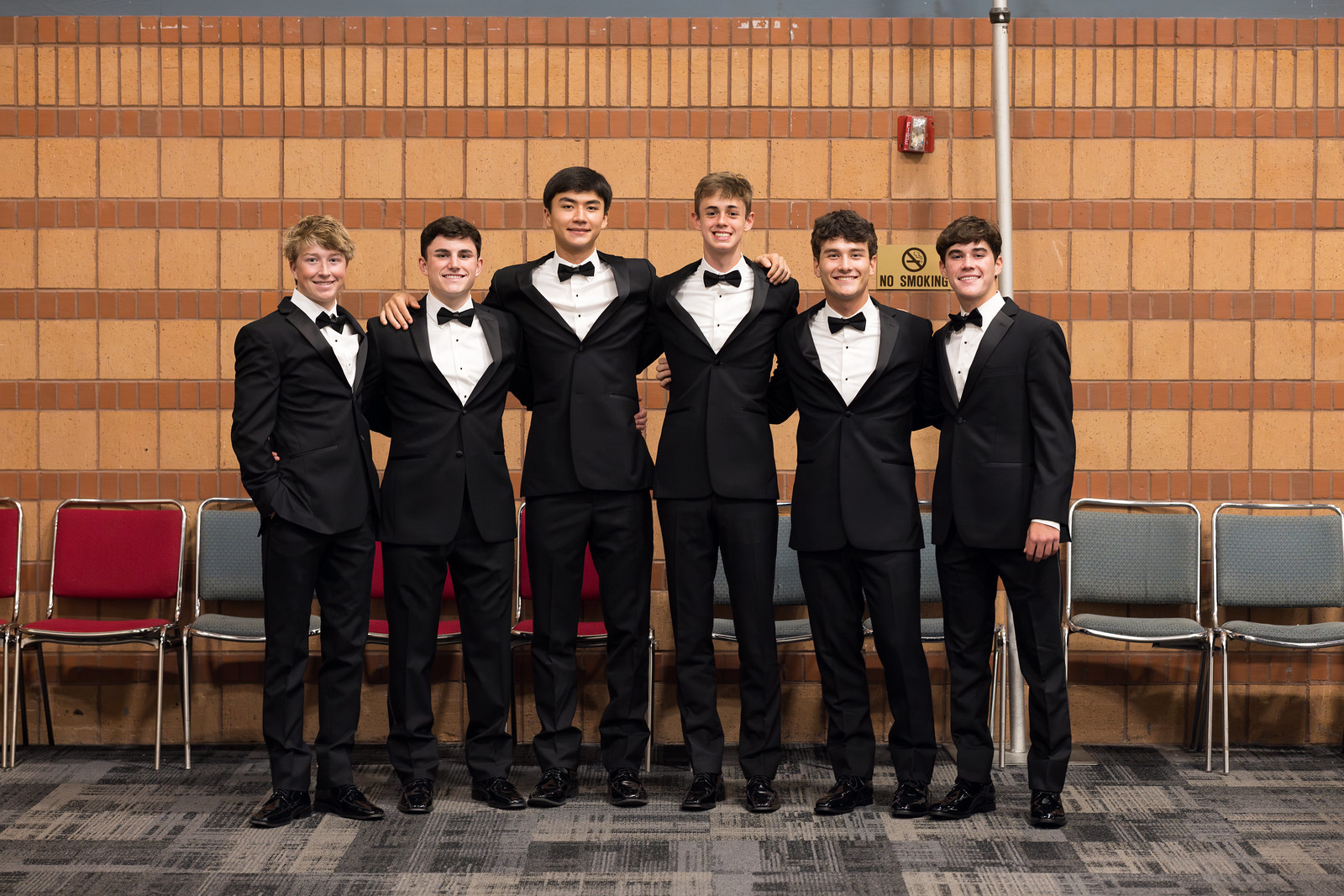In this color photograph, a group of six young men are gathered together, smiling warmly at the camera. They are all wearing black tuxedos with white shirts and black bow ties, perfect for a formal event. Their shiny black dress shoes complete their polished looks. The friends stand in a line, arms draped around each other's shoulders, with the shorter men positioned on the outer edges and the taller ones in the center. They are positioned in front of an array of metal chairs with red and gray cushions. The backdrop features a tan and red brick wall adorned with a "No Smoking" sign and a fire alarm. Below them is a grayish patchwork rug, adding to the casual yet organized setting. The scene hints at a school or community band room, contributing to the overall joyous and cohesive spirit captured in the photograph.